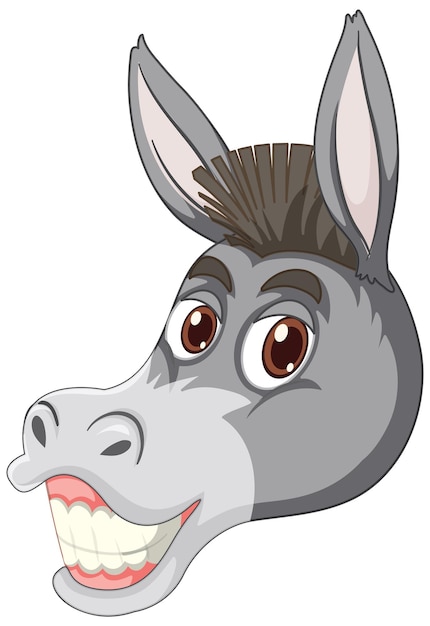This image features a highly expressive, cartoon-style donkey head rendered against a white background. The donkey, characterized by its strangely humanized features, has large, dark brown eyes that look directly at the viewer with a wide, almost exaggerated smile displaying cream-colored, human-like teeth and pink gums. The head is primarily dark gray with a lighter gray muzzle and prominently displays tall ears that stick straight up. Additionally, it sports a mohawk-like tuft of hair between its expressive eyebrows, which cast visible shadows, enhancing its animated appearance. With its anthropomorphic qualities and bold color contrasts, this cartoon donkey exudes a quirky charm.